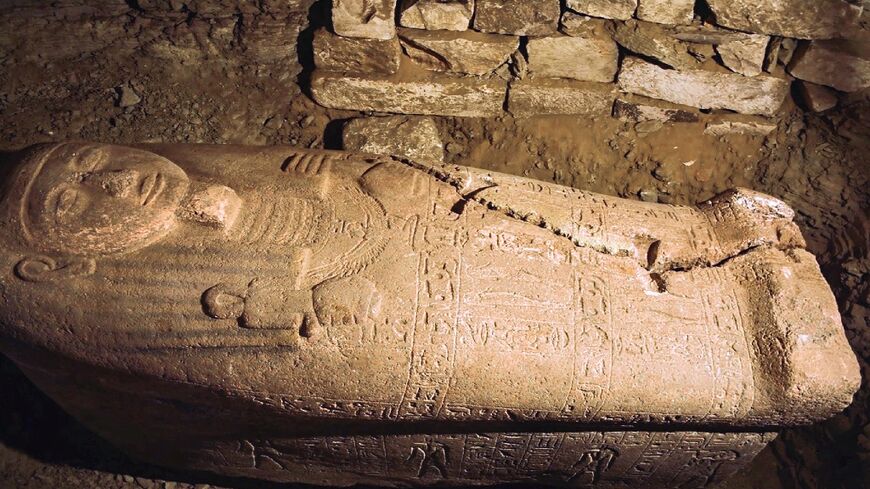The image is a color photograph taken from a high, 45-degree angle, positioning the viewer as though they are standing before an ancient Egyptian sarcophagus. The head of the sarcophagus, adorned with an intricately carved face and traditional headdress, is slightly cut off on the left side, while the feet are on the right. The sarcophagus, which appears to be carved from stone, bears numerous hieroglyphics and detailed patterns across its surface, including a grid-like design around the leg area. A significant crack runs from the middle back to between the feet, hinting at ancient repair attempts, possibly using now-rotted wooden dovetail joints.

The sarcophagus is lying on a raised platform, heavily shadowed but discernible through notches and carvings that suggest it could be made of stone or wood. The surrounding area looks freshly excavated, littered with earth, rubble, and various old stone blocks in shades of brown, cream, and white. Behind the sarcophagus, a background of loosely stacked brick walls adds to the historical ambiance, emphasizing the site's ancient and archaeological nature.

The sarcophagus itself is elaborate, with a detailed carving of a face complete with ears, a long beard, and stripes in the headgear. The arms of the figure are intricately crossed over the chest, with the right hand possibly holding an ankh, a symbol of life, while the left hand clutches an unidentified object. Despite the damage and the large crack, the craftsmanship of the stone sarcophagus remains evident, capturing the essence of ancient Egyptian funerary art.